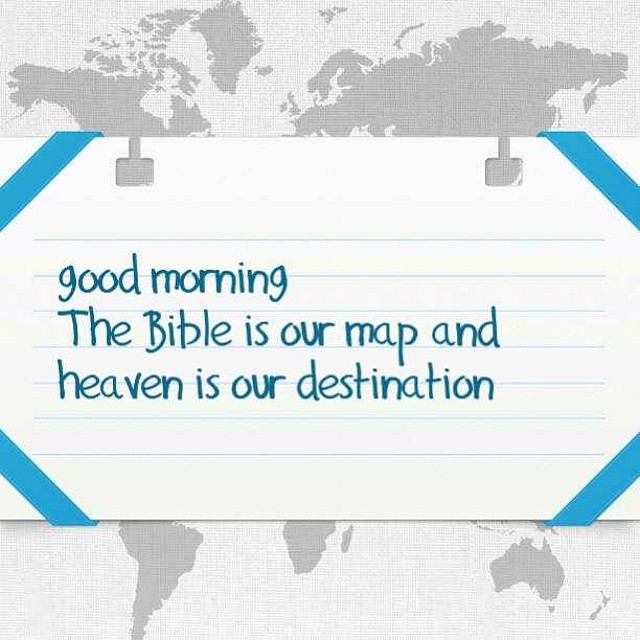The image displays a world map in gray and white as the background. Superimposed on this map is a white sheet of paper with handwritten text. The paper is styled like a card from a Rolodex, featuring blue bands that stretch across each corner. The text on the paper reads, "Good morning, the Bible is our map and heaven is our destination," written in bluish-green letters on horizontal lines. Additionally, there are gray stripes behind the text, adding a layered effect to the visual.